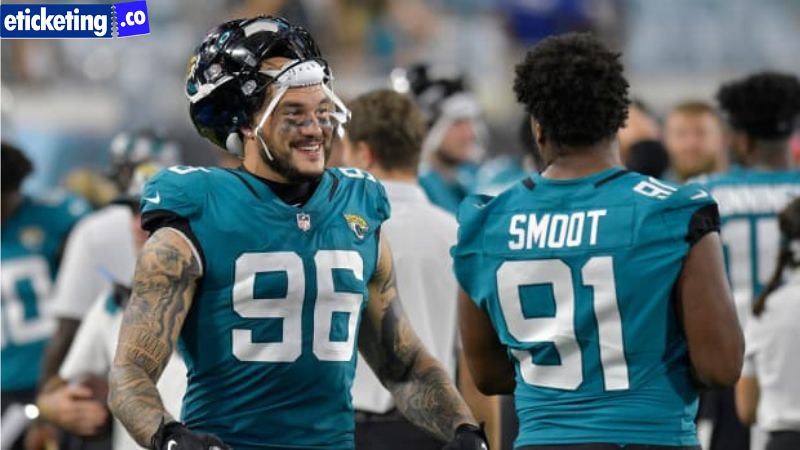In this vibrant snapshot from an NFL football game, the atmosphere suggests it is either pregame or postgame, as evidenced by the relaxed demeanor of the players in the background. Many of them have removed their helmets, while a few still balance them casually on their heads. The photo centers around two main players. On the left stands a white player with extensive sleeve tattoos; his helmet rests atop his head, revealing his bearded face adorned with eye black. He is captured in a moment of joy, smiling warmly at his companion. This companion is a black player, number 91, identifiable by his jersey although he is not in full gear. His smooth black hair frames his face as he looks towards number 96, appearing to be engaged in a pleasant conversation. The camaraderie and relaxed mood of the players give a glimpse into the human side of these professional athletes amidst the bustling game environment.